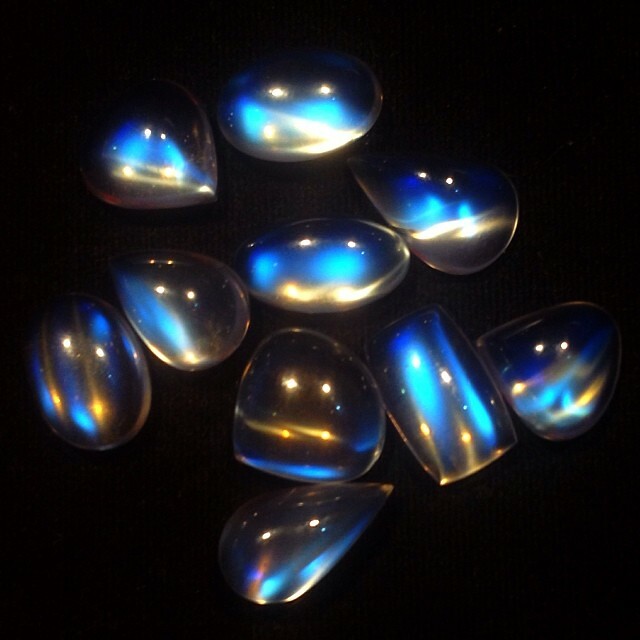The image displays a close-up of nine reflective jewels against a jet-black background, showcasing a variety of intriguing shapes. These smooth, glass-like or metallic objects are meticulously arranged into three rows—two in the top row, four in the second, and three in the bottom row. The objects exhibit a spectrum of colors including light blue, dark blue, gold, and hints of white and black, creating a prismatic effect as the light reflects off their surfaces. The jewels comprise various forms: ovals, teardrops, rectangles, and unique shapes like a heart with a pointed tip and a curvy, rectangular figure. Notably, the central object in the top row is nearly spherical, prominently reflecting dual white lights at the top, with descending hues of blue and gold. To its left and right, the objects take on more elongated, teardrop shapes. The largest item resides in the bottom row. Each jewel’s light reflection varies, enhancing their distinct contours and rich spectrum of colors.